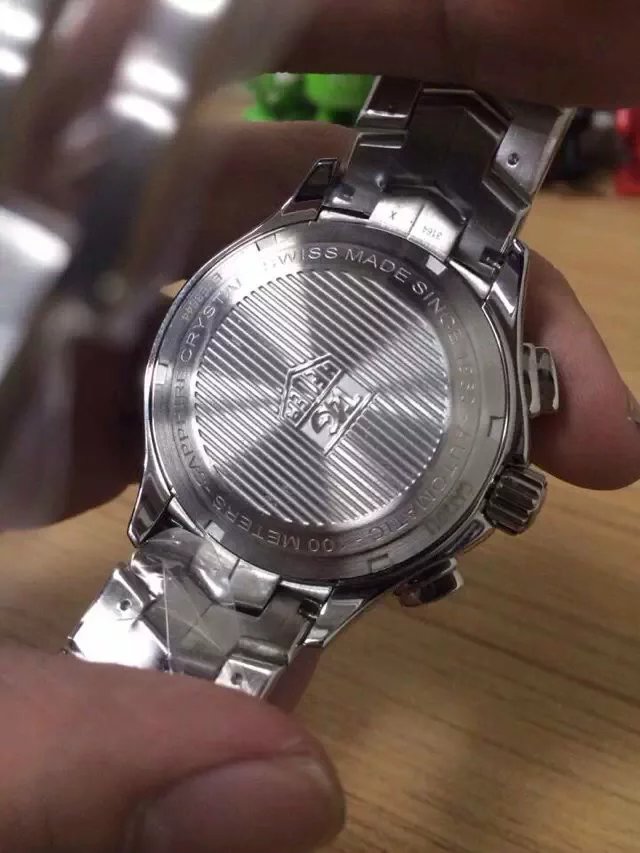In this detailed image, a person's left hand is seen holding the back of a high-end Tag Heuer watch. The thumb is securing the bottom of the strap while the index finger supports it from behind the top. The watch's back features a silver, stainless steel finish with an inscription indicating "Swiss Made" and additional text that is partially obscured by glare but includes the phrases "Automatic," "Sapphire Crystal," and "Meters." The notable Tag Heuer emblem is centered prominently. The watch appears new, with some plastic film still visible on the bottom part of the strap. Also visible are three adjustment knobs on the right side, which are typical for this brand. The backdrop features a hint of greenery, possibly a plant, and the person's thumb rests atop a wood-like surface, likely a table.